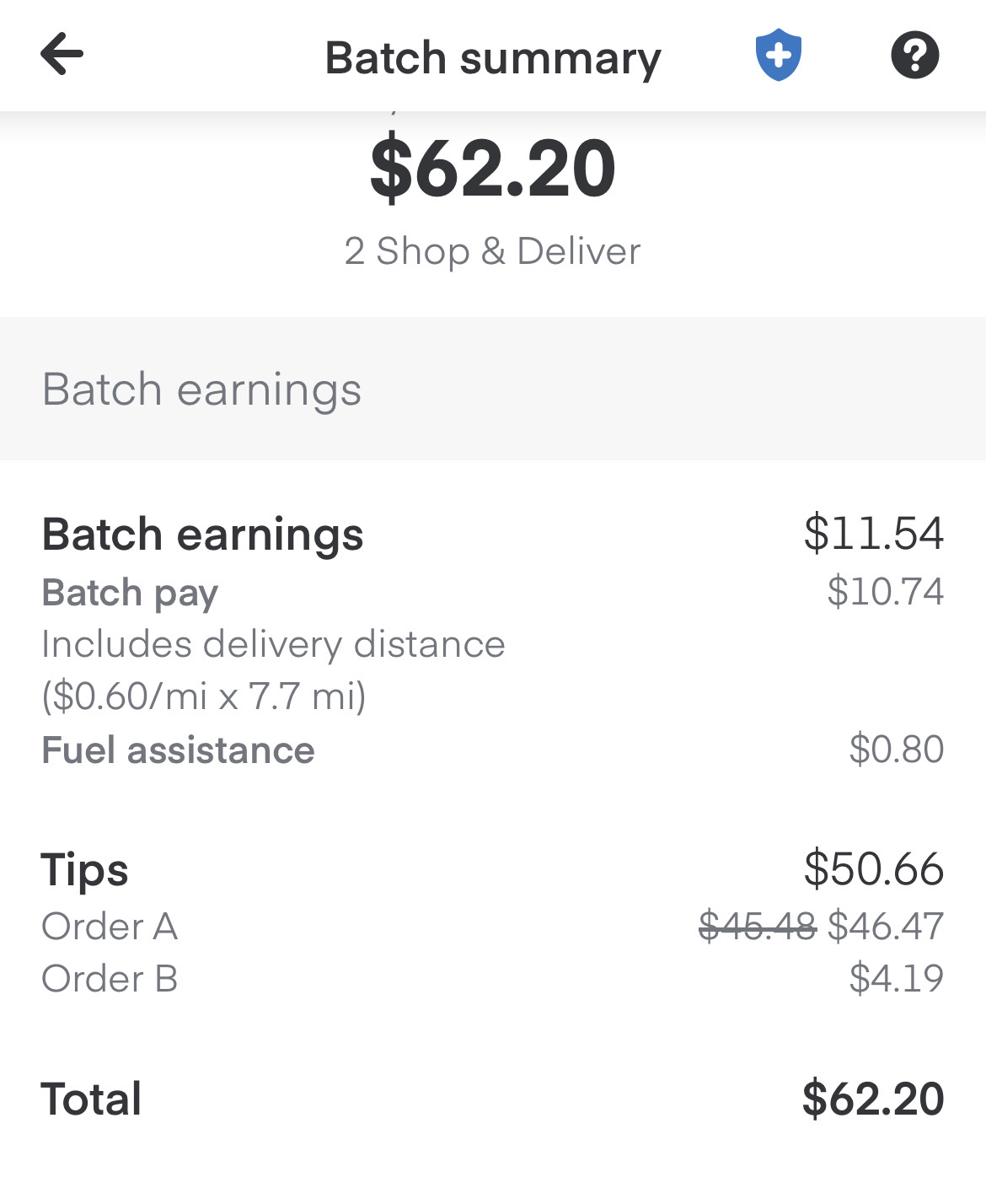The screenshot displays a "Batch Summary" page, which is prominently titled at the top. On the top left corner, there is a back arrow, while the top right corner features a white question mark enclosed within a black circle. Below the "Batch Summary" title, large black text announces the total amount of $60.20. 

Underneath this amount, gray text indicates "To Shop and Deliver". Following this, a detailed list of "Batch Earnings" is presented, organized into two columns: the left column contains descriptive text, while the right column displays corresponding numerical values.

The breakdown of batch earnings is as follows:
- **Batch Earnings**: $11.54
- **Batch Pay**: $10.74 
  (This includes delivery distance calculated as $0.60 per mile for 7.7 miles)
- **Fuel Assistance**: $0.80
- **Tips**: $50.66 
  (Further broken down into Order A: $46.47 and Order B: $4.19)

The overall total tallies up to $62.20.